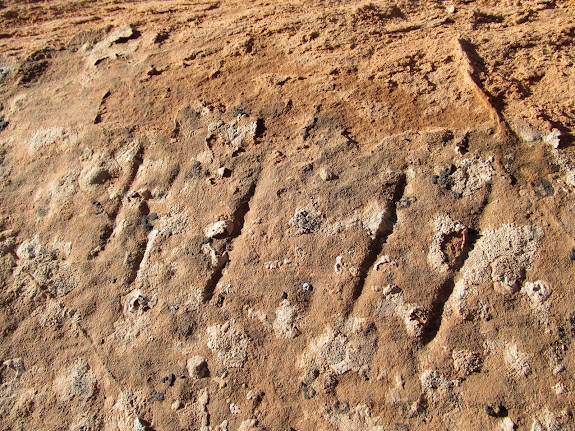This image captures a rugged outdoor scene resembling a Martian landscape with deeply etched lines in the soil. The foreground showcases light brown, uneven soil with small bumps, potentially from dried water deposits. The ground is interspersed with several white mineral patches, suggesting a dry, desolate environment. 

Five prominent lines, possibly drawn with a stick, angle slightly upwards from the left and converge towards the center, forming faint patterns across the dirt. Notably, a thin line in the lower left corner creates a small triangle with the corner of the image, adding a geometrical element to the chaotic terrain.

The colors range from rust-orange to darker and light browns, alongside off-white patches, creating a stark, contrasting palette. The picture, likely taken during the daytime, offers a close-up view of what could be mistaken for the surface of Mars – a reddish, broken, and seemingly otherworldly dirt field.